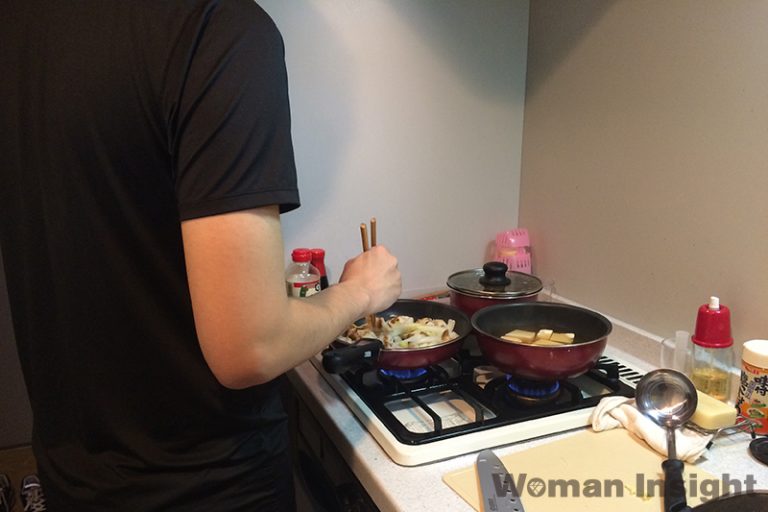A person is cooking in a cozy kitchen setup. Positioned on the left-hand side of the image, they are clad in a short-sleeved black t-shirt and dark pants. The individual is preparing a meal against a white countertop that houses a gas stove with black burner plates. They are using chopsticks to stir-fry contents in a frying pan located on the bottom left burner. Additionally, there is a saucepan with a lid on the top left back burner and another pot on the right-hand burner.

The backdrop includes a cream-colored wall to their left and a beige-colored wall directly in front of them, creating a corner view of the room. On the countertop's left side, a bottle of soy sauce and another unidentified bottle are visible. A pink object sits on the counter in the corner.

The white countertop also features a chopping block situated in the bottom right corner of the image, holding a sharp knife. Nearby, a ladle rests on a dishcloth. An oil bottle and a salt container complete the scene. Overimposed in the bottom right corner of the image are the words, "Woman in Sight."